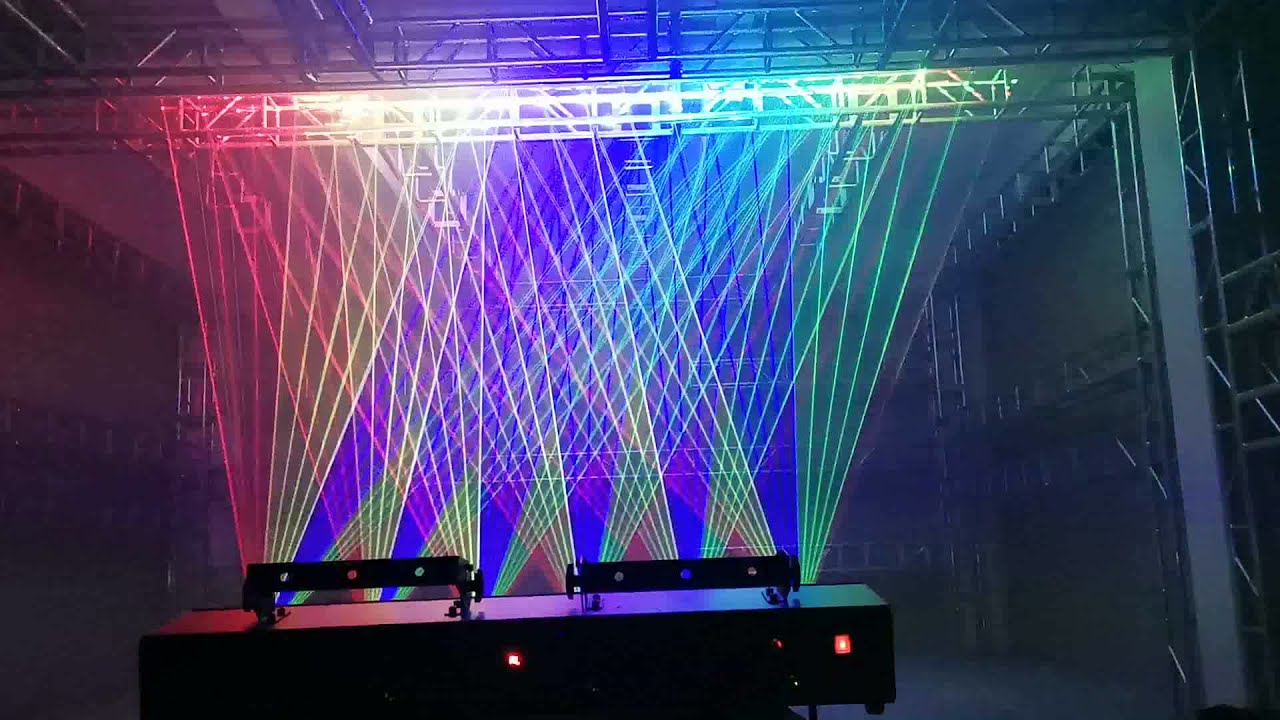The image captures an electrifying scene of a laser light show, possibly taken at a rock concert or a sound stage. At the forefront stands a long, rectangular black machine, reminiscent of an electric piano's rear. Its surface features small brackets and two red buttons, one positioned centrally and the other on the right. The base of the machine is slightly obscured, suggesting it stands on legs. Emanating from this device are numerous tightly focused laser beams, arranged in fan-like configurations. These beams span the color spectrum from red and yellow to purple, blue, green, and white, creating a mesmerizing rainbow effect. In the background, the room is shrouded in darkness, punctuated by steel scaffolding or shelving structures rising about 20 feet high. The overall atmosphere evokes the industrial setting of a warehouse or a sound stage, with the vibrant lasers as the focal point against the stark, shadowy backdrop.